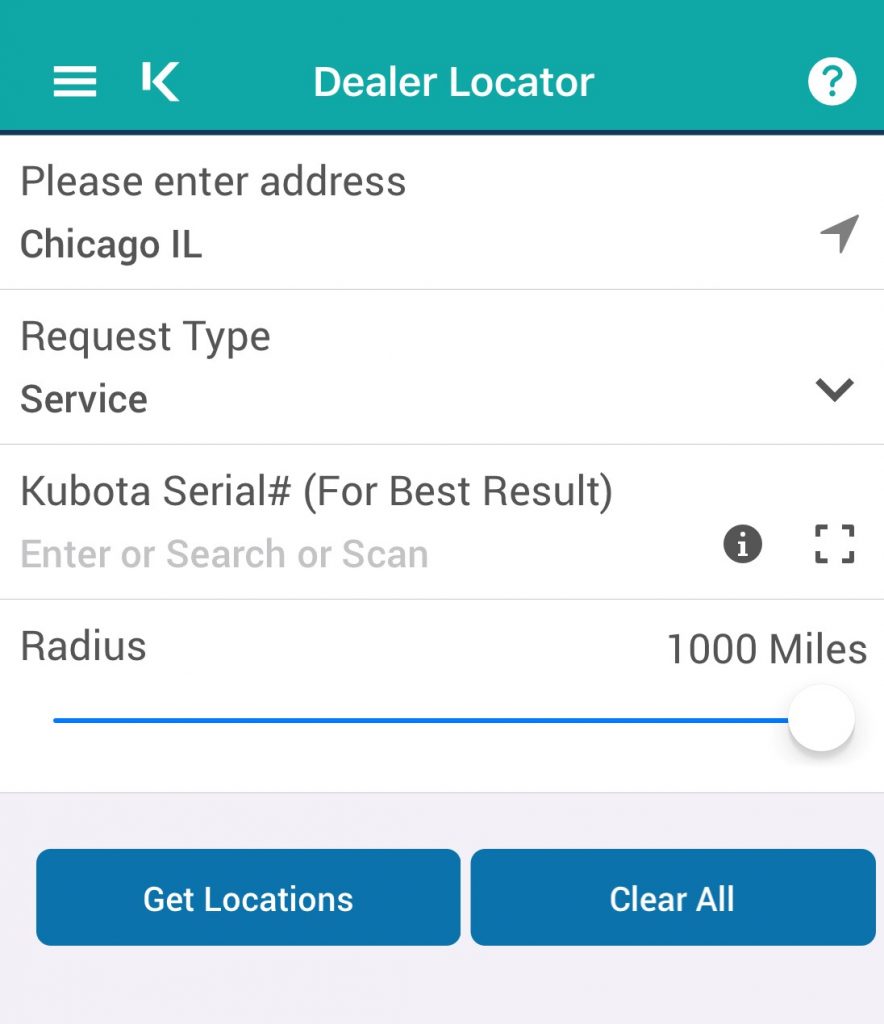The image features a detailed interface layout for a "Dealer Locator" tool. 

At the upper-left corner, there is a light-colored border with a white "K" and three lines, symbolizing a logo or icon. In the middle, the text "Dealer Locator" is displayed prominently. In the upper-right corner, a white circle with a question mark inside indicates a help or information section.

This section is separated by a dark navy blue line, beneath which the background turns white. On the left-hand side, "Please Enter Address" is written in dark gray, followed by the entry "Chicago, IL." A thin gray line divides this section from the next, which is labeled "Request Type" and shows "Service" underneath. Another thin gray line separates this from the section that reads "Kubota Serial," followed by a hashtag in parentheses and an instruction, "For best result, enter or search or scan," in light gray text.

Another thin gray line appears below this instruction, followed by the prompt "Radius." A blue line runs across this section, ending in a white circle on the right side.

On the left-hand side, there are several controls: at the first level, a gray arrow pointing up; on the second level, an arrow pointing down; on the third level, a gray circle with an "i" inside, forming part of an outlined square. On the last row, "1,000 miles" is displayed.

At the bottom of the interface, there are two blue tabs against a gray background. The first tab, in white text, says "Get Location," and the second one says "Clear All."